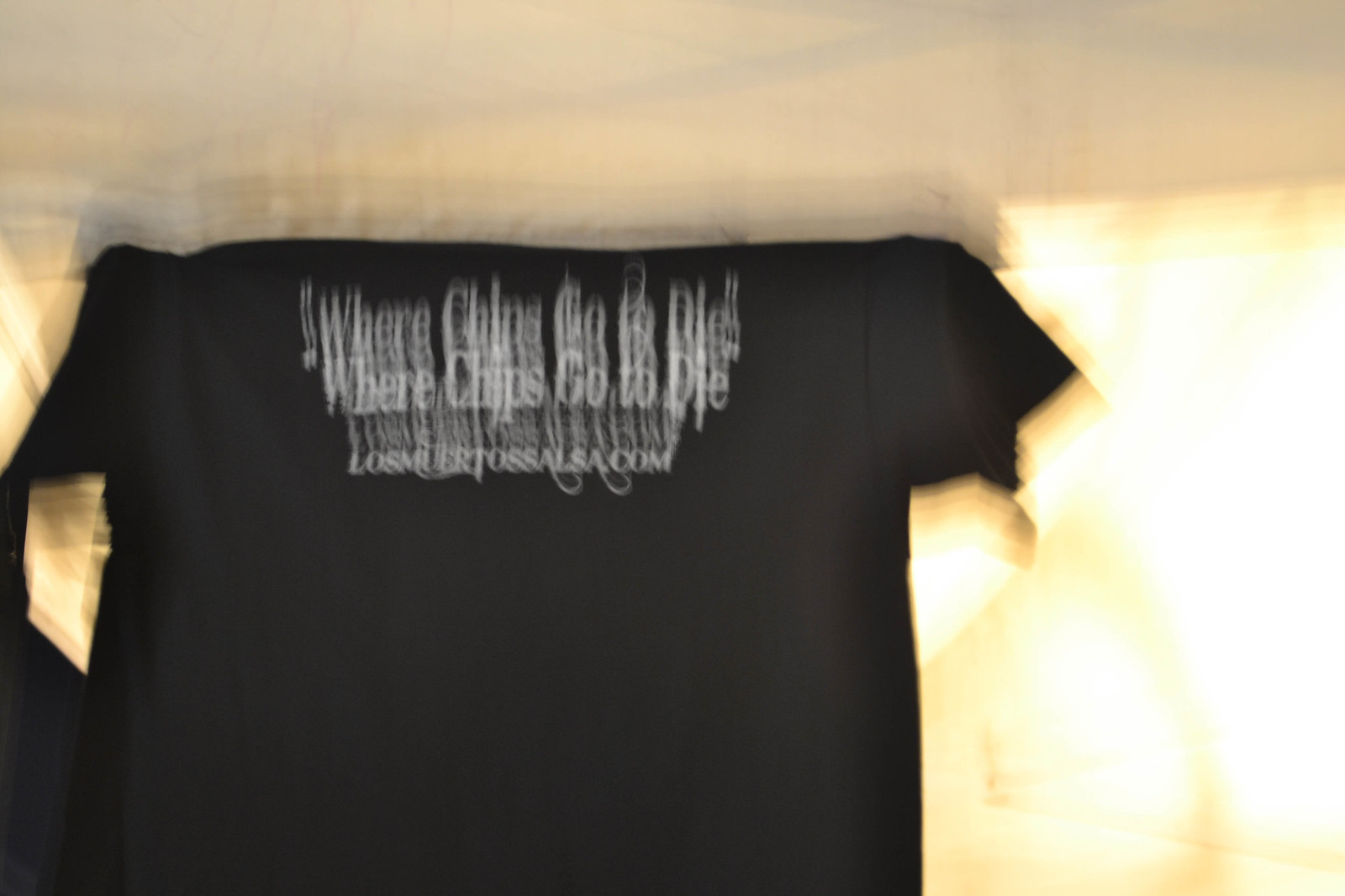The image depicts a black t-shirt with obscure and somewhat disorienting lighting, making it challenging to ascertain if it is being worn by someone. The shirt prominently displays a quotation in doubled, slightly blurry white font that reads, "Where chips go to die." Below the quote, there is a URL, "lasmirtosala.com," suggesting a promotional aspect for a website, though its purpose remains unclear from the image alone. The peculiar doubling of the text implies that the photograph might have been taken mid-movement, adding to the off-kilter, almost ghostly appearance of the words.